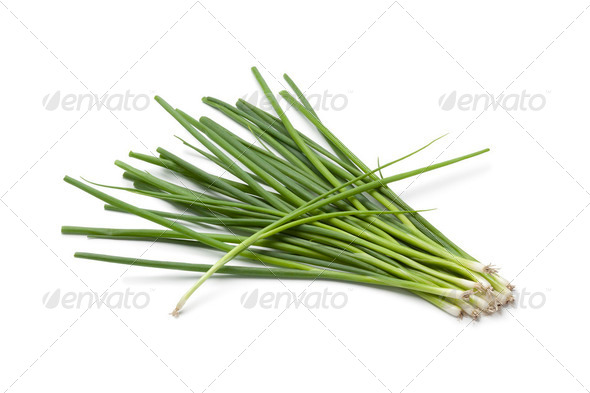The image depicts a meticulously arranged bunch of about 10 to 12 green onions, also known as scallions, lying on a white background with a subtle gray grid pattern and an embossed logo featuring the brand name Envato alongside a stylized leaf design. The green onions are oriented with their white bulbous roots on the right and their long, dark green leaves extending to the top left, except for one individual stalk that lies crosswise on top of the rest of the bunch. The arrangement casts soft shadows on the plain white surface, further highlighting the fresh, vibrant green to white gradient of the onions.